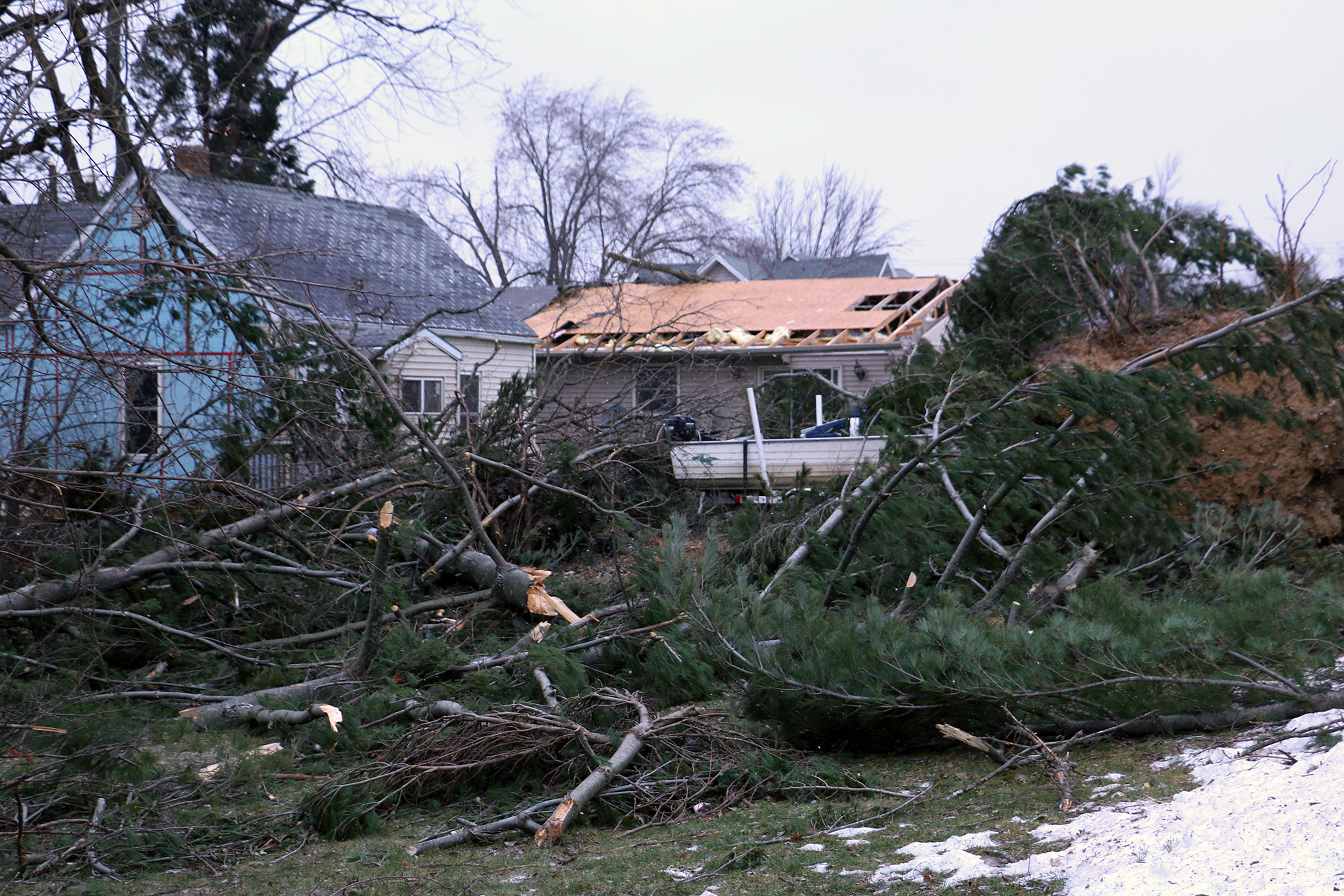The image captures a scene of extensive destruction outside, seemingly caused by a tornado. In the foreground, freshly broken tree branches are scattered right and left across a yard, their light-colored interiors clearly visible. To the right, a mound of dirt suggests the fallen tree's origin. There is a light dusting of snow on the lower right side, indicating cold weather conditions. Two houses are prominently featured in the background: the one on the left has sustained significant damage with a partially missing roof, exposing the bare wood and interior holes. Behind it, another house also shows signs of roof damage but to a lesser extent. On the far right in front of the damaged houses, part of a boat hull is visible. The sky above is gray, adding to the overall somber mood of the scene. The colors in the image include shades of green from the trees, white from the snow and exposed roofs, as well as patches of blue, tan, and brown throughout.